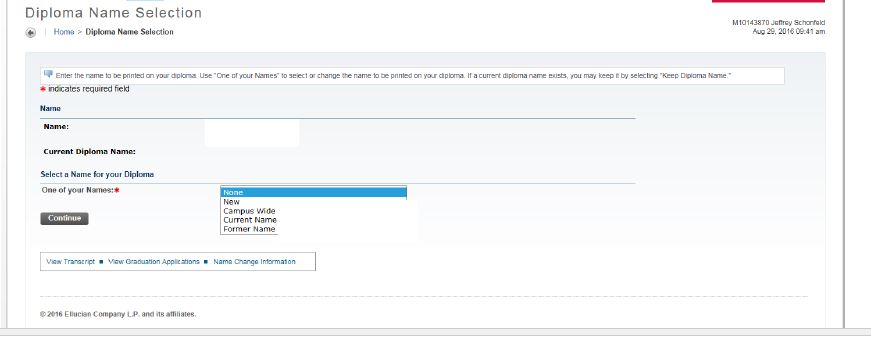Screenshot of Diploma Name Selection Interface - Dated August 20, 2016

The screenshot showcases a user interface pertaining to the selection of a diploma name, featuring the name Jeffrey Scharnfeld in the upper right corner, accompanied by an unreadable text and numeric string. This interface, dated August 20, 2016, includes a visible timestamp that is difficult to decipher. 

The top left of the screen contains a "Back" button, followed by a navigation path: "Home > [Caret] > [Submenu]". This indicates that the user is within a diploma name selection submenu. Below this navigation area lies a large textual field, which appears to provide instructions or information, though its contents are too small and pixelated to read clearly. 

An important field is marked with a red asterisk, signifying it as a required field. This is followed by a section labeled “Current Diploma Name” with an entry field beneath it. Unfortunately, the specifics of this field are unreadable due to the poor image quality.

Further down, the interface prompts the user to “Select a name for your diploma” and provides several options such as "one of your names," "none," "new," "campus-wide" (or “campus video”), "current name," and "former name." However, details about the names available for selection are not visible. 

Below these sections, additional options and resources are listed: "View Transcript," "View Graduation Applications," and "Name Change Information." 

At the very bottom, there is a small, barely legible text indicating the company name and date, likely referenced as "2006 something something Company LP".

Due to the low resolution of the screenshot, a higher quality or larger image would considerably enhance readability and user experience.